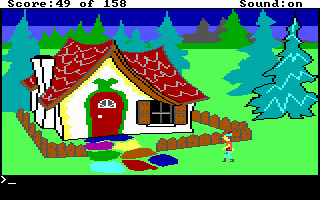This highly pixelated and simplistic screen capture from a children's video game vividly showcases a small, cartoonish white cottage situated on green grassland. The prominent features include a red roof with peculiar sloping sections, a red door adorned with a green eagle-like image above it, and a dark brown picket fence encircling the house. The house has brown shutters and a single window next to a chimney. A multicolored stone pathway—consisting of blue, purple, green, yellow, red, and magenta stones—leads up to the front door. At the top of the screen, the score is displayed as "49 of 158" with the sound being on. In the foreground, a small male figure in a red shirt and green pants stands in front of the fence. The backdrop features numerous large and simple evergreen tree outlines against a sky with two distinct purple and dark blue bars. A black bar with a cursor prompt at the bottom indicates interactive elements of the game.